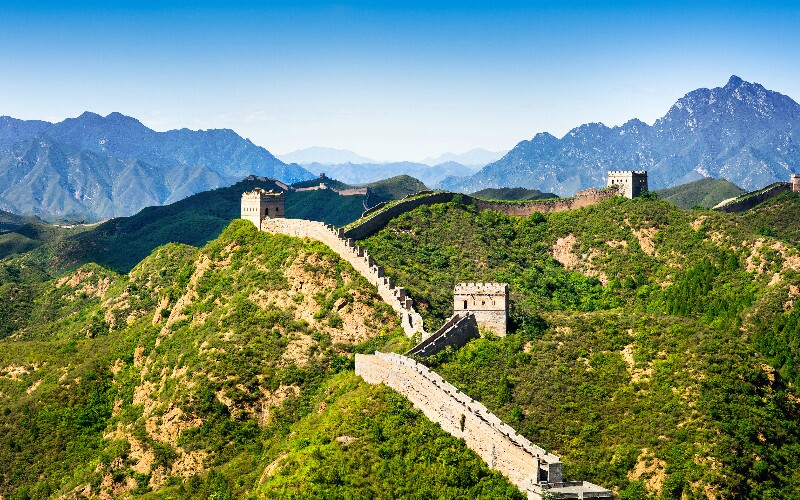This is a detailed photograph of the Great Wall of China, captured outdoors during the daytime. The Great Wall, characterized by its ancient tan, light rock, and cement-like color, extends prominently from the lower right corner of the image. It scales a steep, tan-colored mountainside, and the structure is marked by periodic towers approximately every quarter mile that connect the walkways through the fortifications. At one notable point, the wall branches from the center to both the right and left, leading to fortresses strategically positioned along its path. Surrounding the wall, lush greenery of shrubbery and trees contrasts vividly with the brown hills and tan mountain sides. In the distance, an expansive mountain range composed of black-gray and blue hues provides a dramatic backdrop, with peaks stretching up and forming a dip in between. Above all this, the sky transitions from white to a bright blue, interspersed with occasional clouds just behind the mountain summits. The dimensions of the photograph are approximately 6 inches wide by 3 to 4 inches high, capturing an extensive and picturesque view of this historic site.